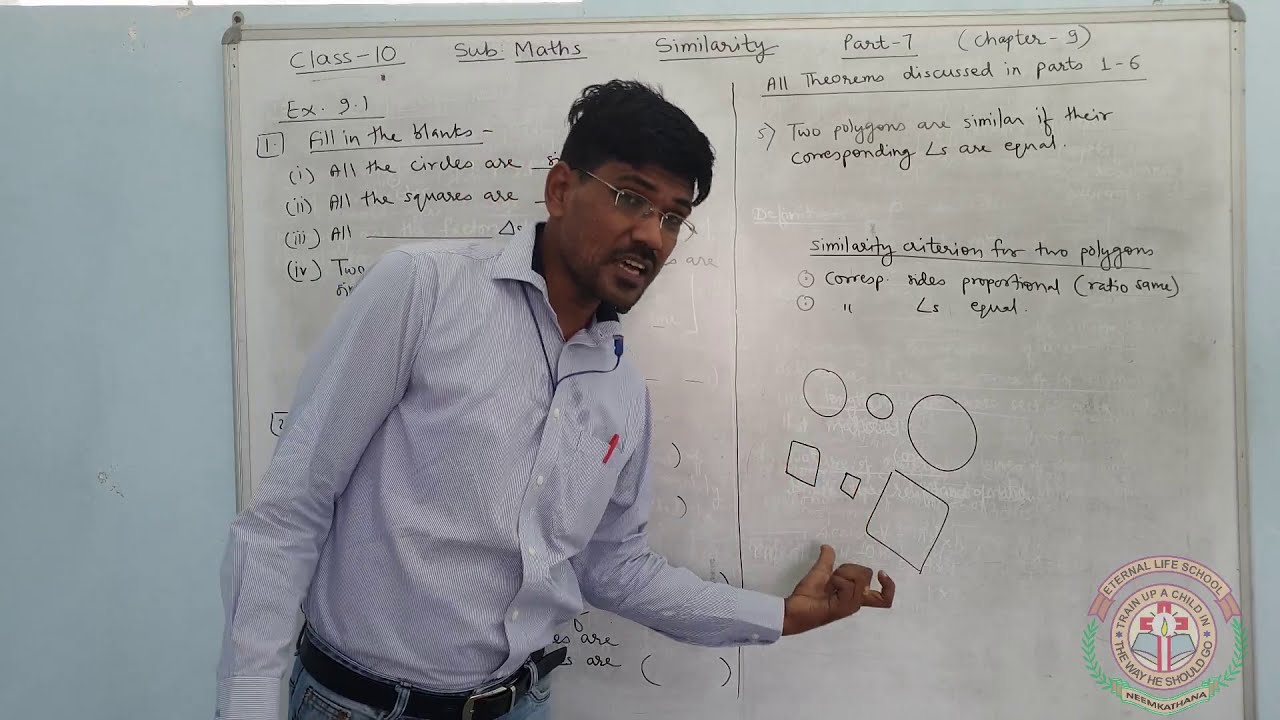The image features a male, approximately between 25 to 30 years old, who appears to be a professor conducting a presentation at the front of a classroom. He is situated in front of a dirty whiteboard mounted on a light pastel blue wall. This whiteboard, marred by remnants of previous writings, showcases numerous texts and diagrams including references to circles, squares, theorems, and a mix of mathematical notations and instructional phrases like "class IO," "sub," "math similarity," and "part seven, chapter nine." Some of this content is partially obscured by the professor himself. 

He is actively engaging with the material, gesturing with outstretched hands towards various elements on the board. The professor is dressed in a light blue long-sleeved collared shirt that is tucked into dark blue jeans, secured with a black belt. His appearance is characterized by dark skin, dark hair, and thin silver wire-rimmed glasses, with a slight beard and mustache. He is speaking, as evidenced by his slightly open mouth, and possibly wears a lapel microphone to aid his presentation.

In the lower right corner of the image, there is a transparent, multicolored logo consisting of light green, peach, and soft red elements. The logo depicts a book, a cross, and a lit candle, accompanied by the text "Eternal Life School" and the motto "Train up a child in the way he should go."